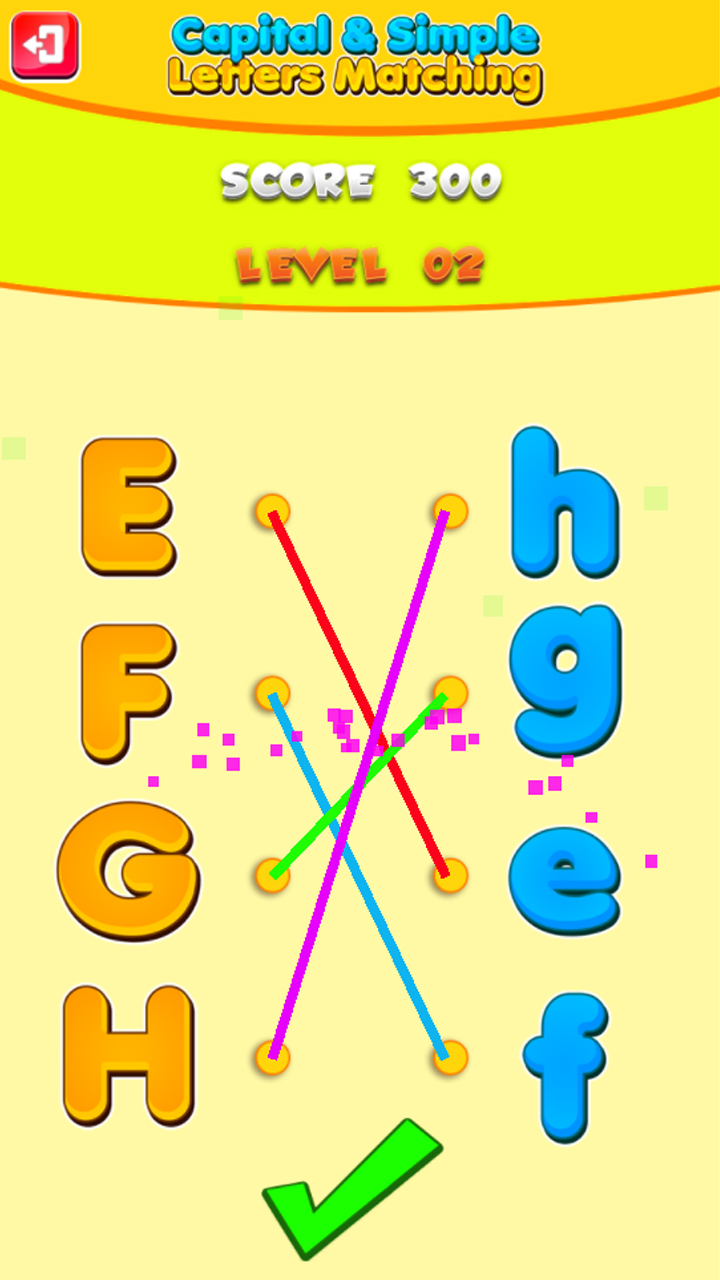This screenshot depicts a children's educational mobile game designed to teach letter matching. The game's interface features a clear and engaging layout suitable for young learners.

At the top, blue text prominently displays "Capital and Simple," indicating the game's focus on letter case matching. Below this, the title "Letters Matching" appears in bold orange text with a semicircular orange design curving underneath.

In the top-left corner, a red "Exit" icon with a stick figure exiting a doorway signifies the option to leave or navigate out of the game. Just beneath this icon, white text indicates the player's current score, which is 300. Below the score, dark orange text displays the current level, noted as "Level 2."

The main game screen presents an interactive matching activity where players connect uppercase letters on the left to their corresponding lowercase letters on the right. The uppercase letters are displayed in orange, with "E" at the top, while the lowercase letters are in blue, with "e" positioned third from the top on the right side. Players must draw lines to match each uppercase letter with its lowercase counterpart, creating an engaging and educational activity that promotes letter recognition and learning.